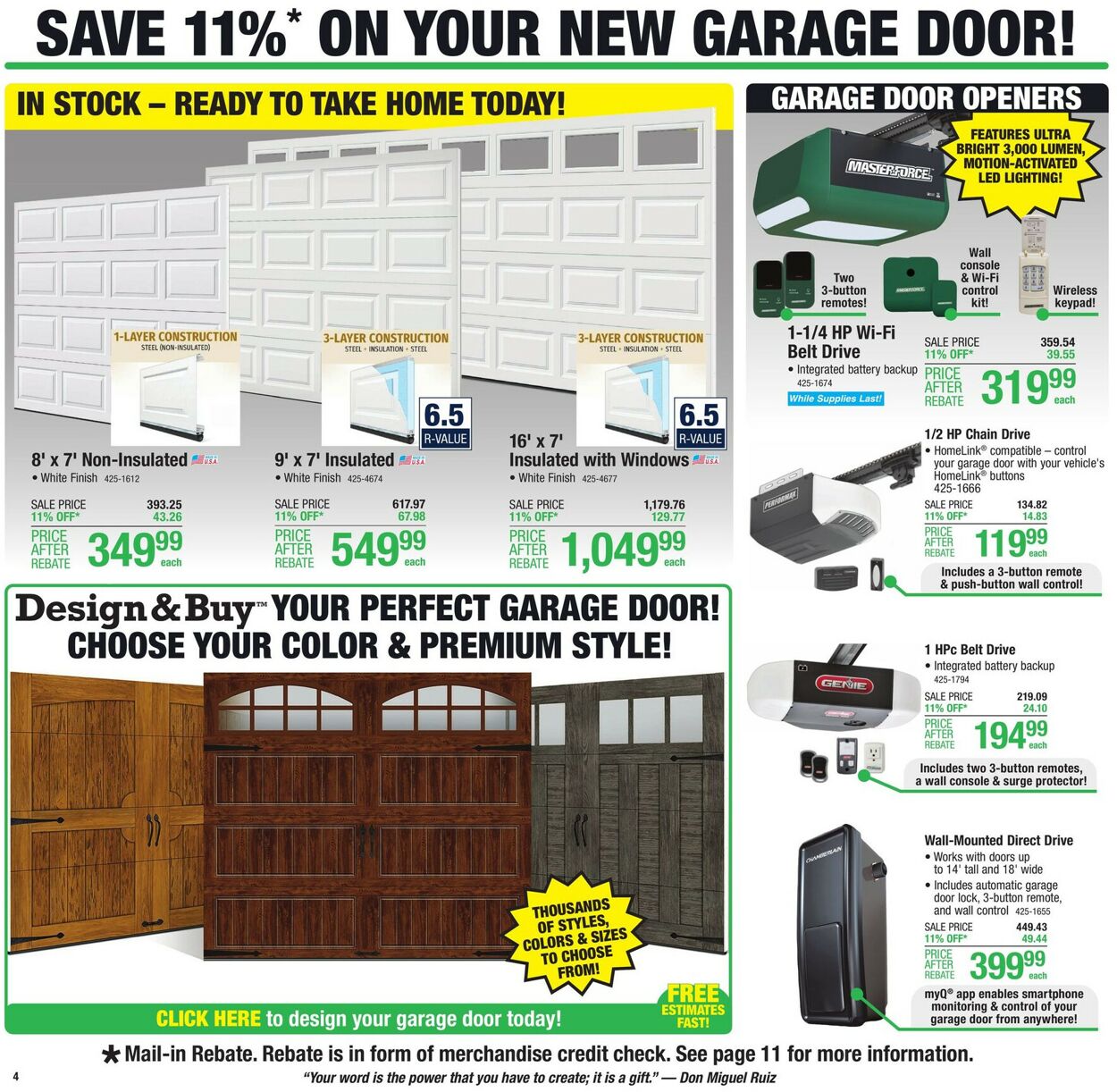Menard's Advertisement: Save 11% on Your New Garage Door! 

Discover great deals on a variety of in-stock garage doors, ready to take home today. Options include traditional white doors for single-car and two-car garages, including two-car models with windows at the top. For a rustic look, choose from beautifully crafted wood options resembling barn doors. 

Design and customize your perfect garage door with a vast selection of thousands of styles, colors, and sizes. Enjoy fast and free estimates to help bring your vision to life.

To the right, explore a range of garage door openers:
- 1.25 HP Wi-Fi Drive Belt Garage Door Opener for $319
- 0.5 HP Chain-Driven Garage Door Opener, including a three-button remote and push-button wall control, for $119
- 1 HP Belt Drive Garage Door Opener for $194
- Wall-Mounted Direct Drive Garage Door Opener, compatible with doors up to 14 and 18 feet wide, featuring an automatic garage door lock, three-button remote, and wall control for $399

Find everything you need to upgrade your garage door at unbeatable prices!